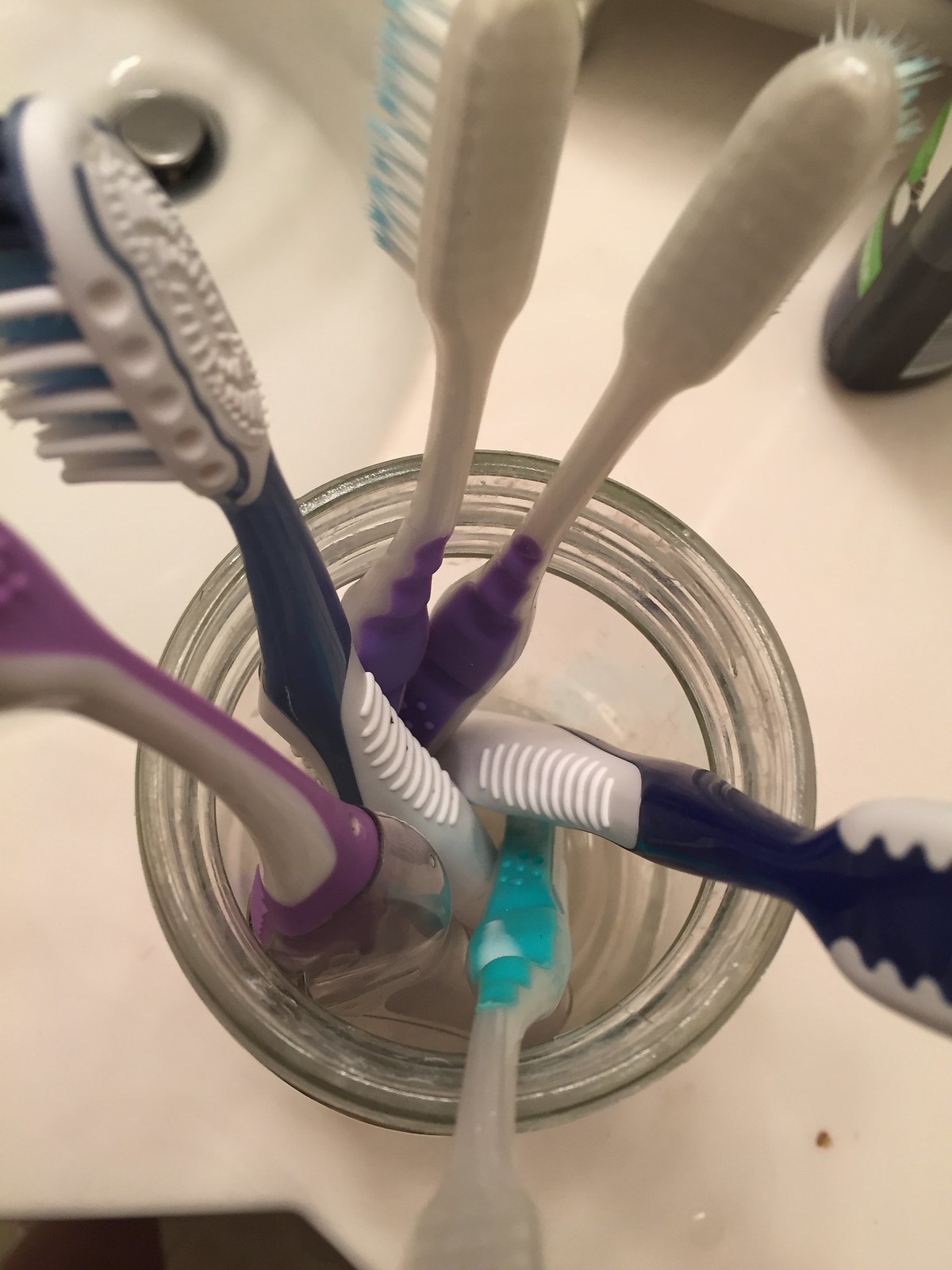The top-down image captures six toothbrushes standing upright in a glass jar positioned on a white bathroom countertop, partially covering a bathroom sink and its visible drain at the top left corner. The toothbrushes exhibit a variety of colors and patterns: two dark blue with white, two purple with white, one turquoise with white on both the handle and brush head, and another partially visible one that appears mostly pink with white. To the top right of the frame, there is a stick of deodorant, though its brand is indeterminate, and a small mark or dirt is noticeable on the bottom right of the countertop. The photo emphasizes the unique and shared color schemes, as some toothbrushes have color extending all the way to the brush head, while others have distinct sections of color on the handles.